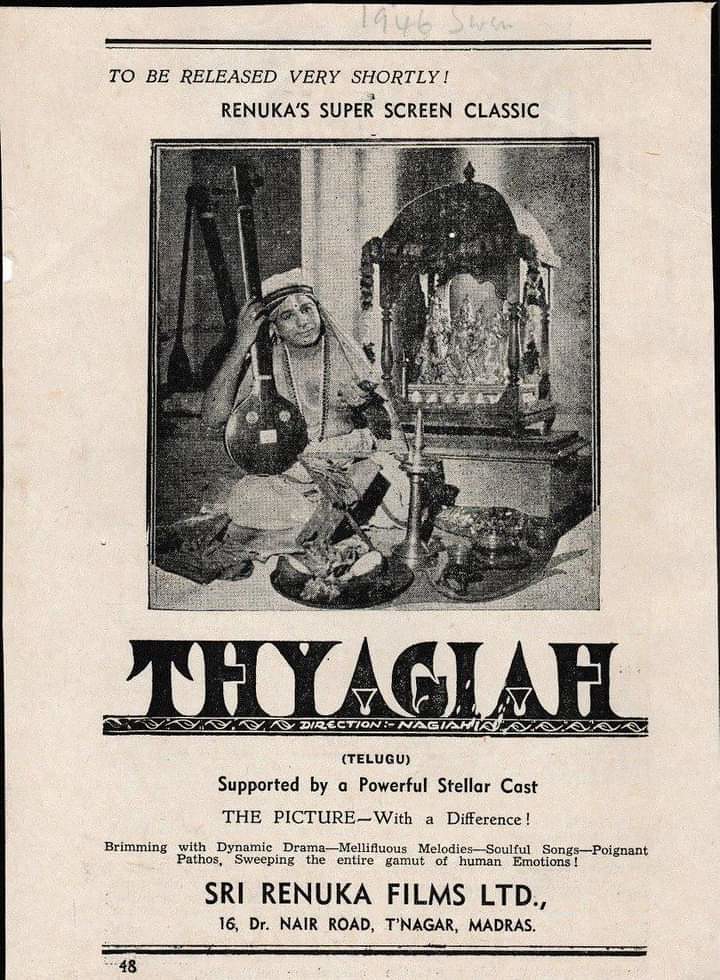The image appears to be an aged, dingy off-white poster or magazine page with faded black print. It features the title "To be released shortly, Ranuka's Super Screen Classic" prominently at the top. At the center of the poster, there's a grainy, black-and-white photograph bordered by a black outline. The photograph depicts a person, possibly a woman, wearing a headscarf with fabric hanging down, adorned with a necklace, and holding a musical instrument on their leg. In the background, a shrine with statues is visible, along with a candle holder and some shiny silverware on the floor in front. Bold and elegant black letters spell out "T-H-Y-A-G-I-A-H" beneath the image, and a black bar with squiggly lines contains the word "Telugu" in parentheses. Further down, the text "supported by a powerful stellar cast" and "a picture with a difference" is noted. The poster also advertises the film as "brimming with dynamic drama, melodious melodies, soulful songs, poignant pathos, sweeping the entire gamut of human emotions." At the bottom, "Sri Ranuka Films LTD, 16 Dr. Nair Road, T. Nagar, Madras" is printed as the address.